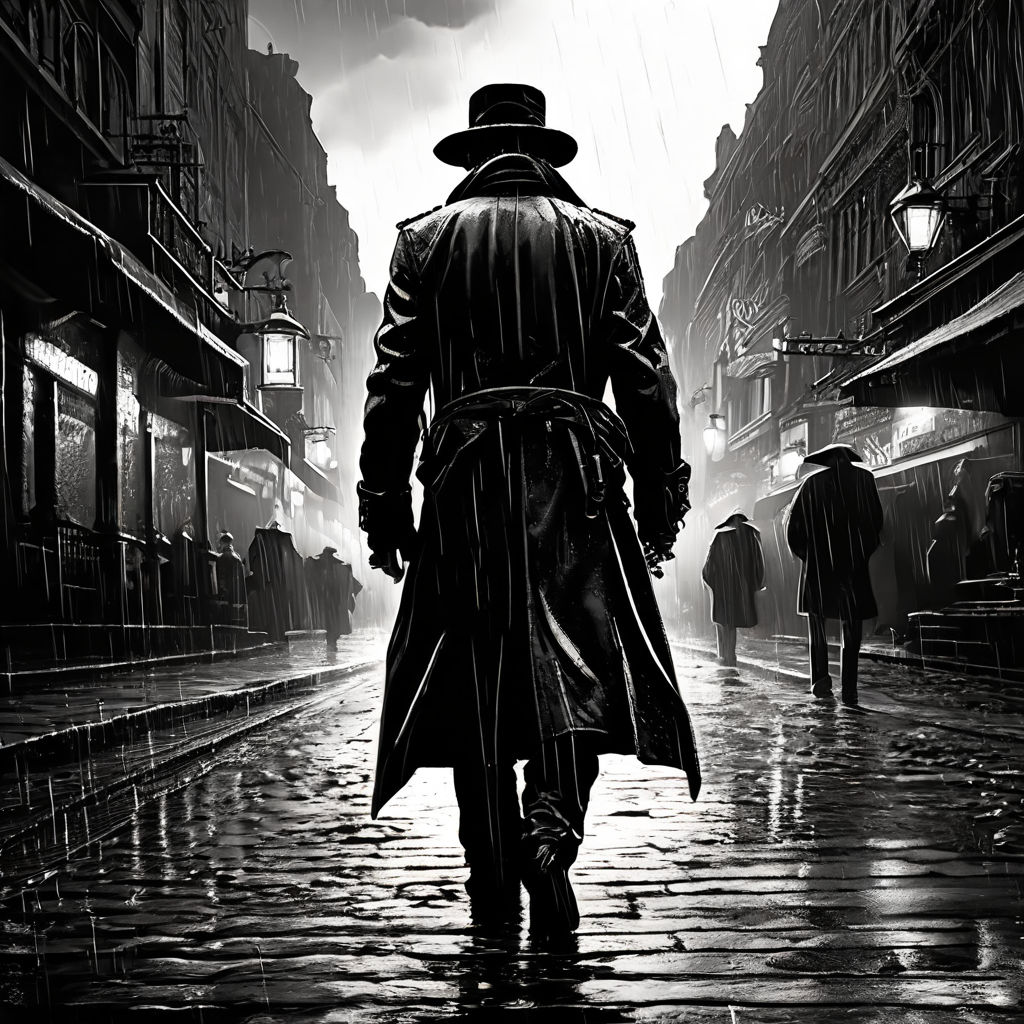This detailed black and white illustration captures a rainy day in a Victorian-esque city. Central to the scene is the back of a man walking down a wet, cobblestone street, illuminated by reflections from the rain. He wears a black trench coat and a hat with a flat brim. Both sides of the street are lined with traditional buildings, some featuring canopies extending from their facades and large, hanging lanterns. The man's direction is mirrored by several other figures, also clad in similar trench coats and hats, who walk ahead of him on the pedestrian pavements. The overcast sky looms gray above, intensifying the somber, rainy atmosphere.